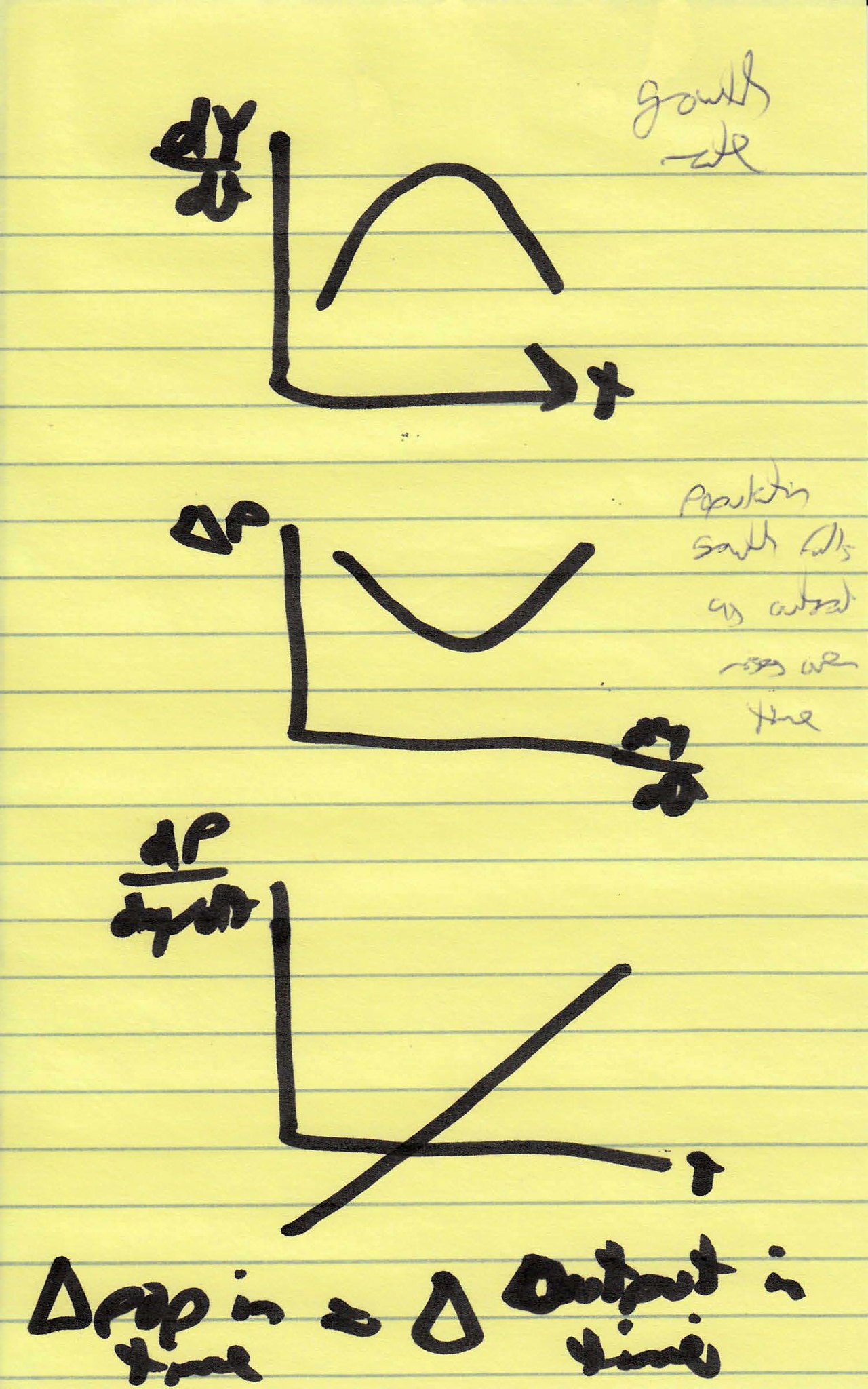This is a portrait-style image on a yellow piece of lined paper, with blue horizontal lines. The paper contains three distinct graphs aligned vertically. 

The first graph, positioned at the top of the image, features an x-axis labeled "x" to the right and a y-axis without a specific label visible here. Inside this graph, a half-circle is depicted with only the upper portion visible. Above the y-axis, "dy" is written, and beneath it, the letter "d" is underlined, all in marker.

The second graph, located in the middle, also has an x-axis labeled "x" to the right and a y-axis with "ΔP" written at its top. This graph contains an upside-down half-circle displaying only its lower part. On the right side of the x-axis, the equation "dy/dx" is indicated.

The bottom graph displays an x-axis labeled "x" to the right and a y-axis with "dP" underlined, followed by "dy/dx" written at its top. A straight diagonal line cuts through this graph, extending halfway through the graph and continuing outside of it. Below the graph, there is a label reading "ΔP," followed by "Δ" and "output in time."

This detailed sketch, annotated with mathematical symbols and equations, appears to convey various mathematical concepts and relationships.